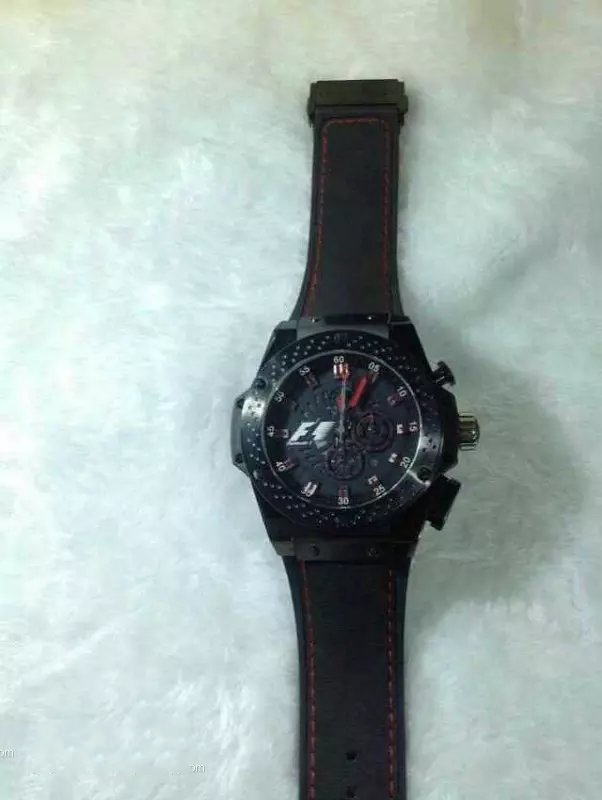This vertical rectangular image showcases a black wristwatch placed on a white marble-like surface with light gray veining. The watch is oriented vertically with the band stretched from the top to the bottom of the frame. While the connecting hardware of the band is not visible, the watch face commands attention. The watch face is entirely black, accented only by the black and red hour and minute hands. Encircling the watch face are numbers in sequential order, starting from the top and proceeding clockwise: 60, 5, 10, 15, 20, 25, 30, 35, 40, 45, 50, 55, and concluding again at 60. Within the main dial, the watch also features two smaller sub-dials, though their purposes aren't clearly discernible due to the image's slight blurriness. These sub-dials potentially serve to measure additional parameters. The overall visual is one of sharp contrast between the dark, intricate details of the watch and the clean, elegant background.